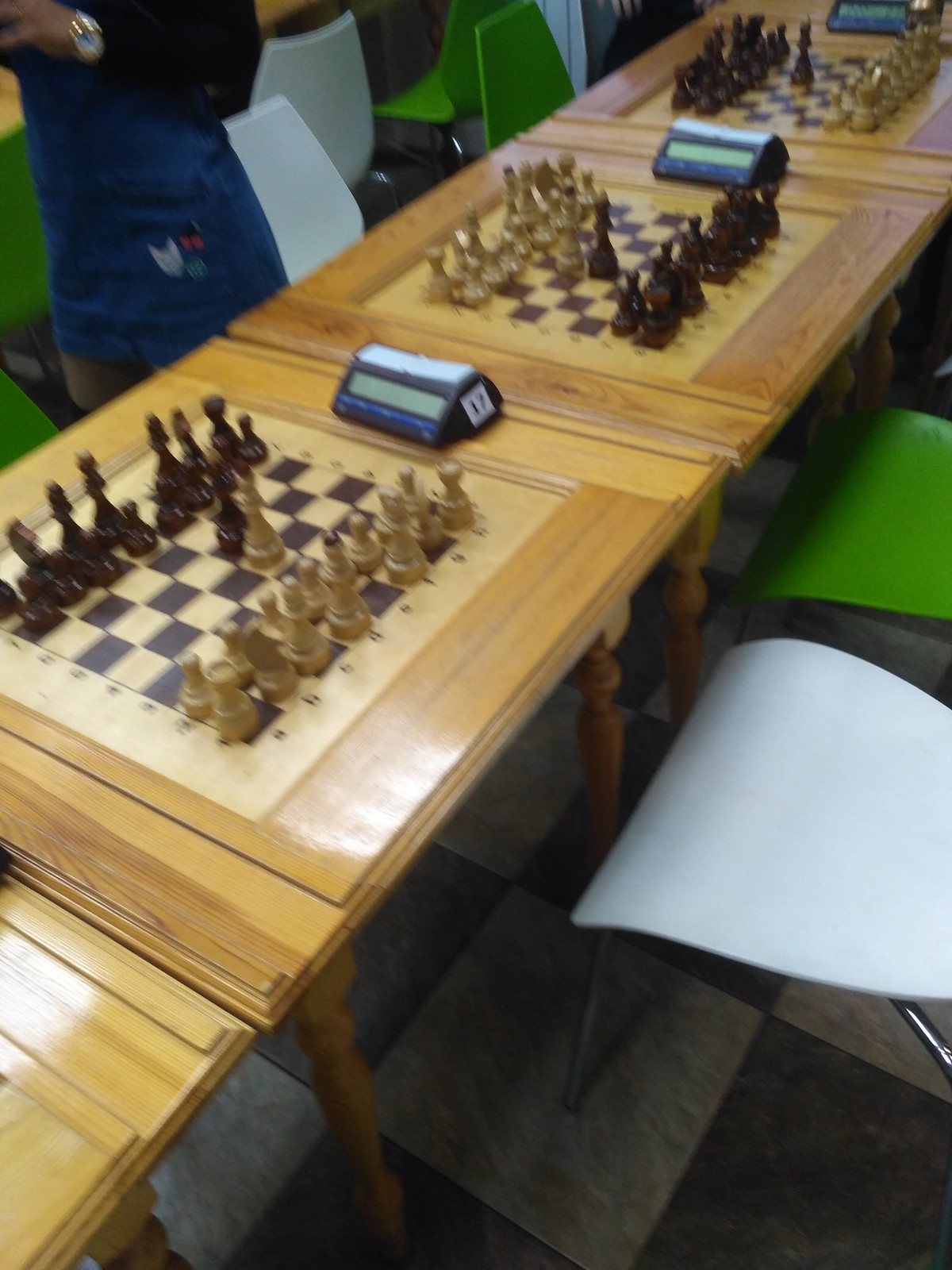The image captures a row of four small wooden tables, each featuring a built-in chess board framed in wood with spindle legs. The chess boards, comprised of light beige and black squares, hold intricately arranged chess pieces in black and tan. Each board has a timer positioned to the right, suggesting an active chess competition. Seated around these tables are pairs of green and white fiberglass-style chairs with metal frames. In the background, at least one or two people, including a Caucasian female wearing a jean dress and a black top, are standing, overseeing the event. Despite the presence of timers and strategic piece placements indicating ongoing games, no one is currently seated and playing. The overall scene suggests a chess tournament setting poised for the next move.